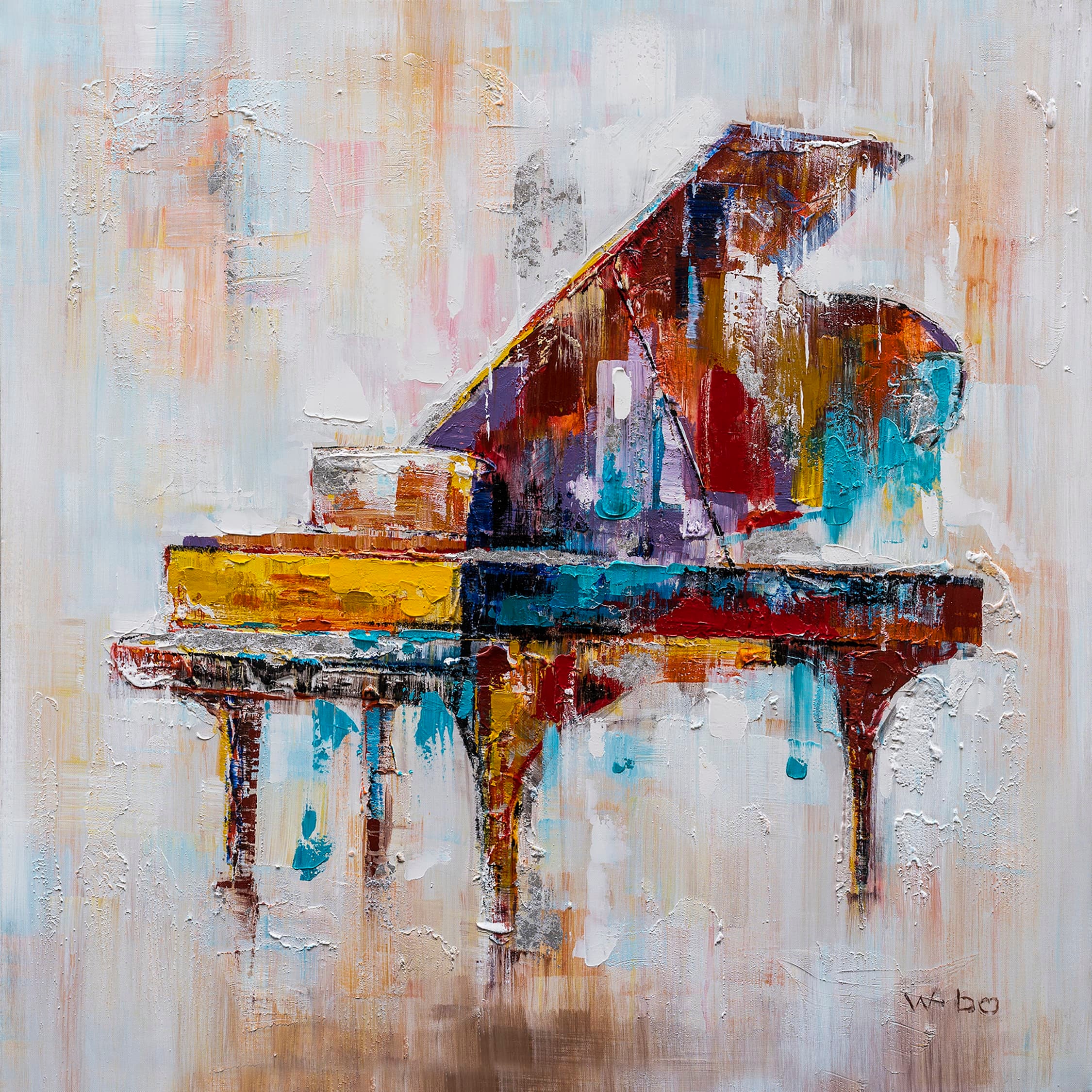The image is an abstract painting featuring a grand piano as the central subject. The piano is depicted in a close-up view with its hood open, revealing a multitude of colors, including reds, dark browns, oranges, and yellows. The edges of the piano are irregular and flow with the paint, giving it a melting, etched appearance. The front panel above the keyboard is prominently yellow, and the keyboard area itself is white with surrounding blue accents. The piano's legs are painted in an array of hues: the far-left leg shows red, white, blue, yellow, and black, while the legs on the right exhibit mixtures of brown, black, and blue.

The background of the painting is textured and rough, filled with light blues, whites, pinks, light oranges, and dark browns. These colors form a dynamic backdrop that contrasts with the piano's vivid colors. Notably, in the bottom right-hand corner of the painting, the initials "WBO" are inscribed, adding a personal touch to the piece. The painting features distinct brush strokes and a textured surface, with paint appearing dry and layered, enhancing the overall abstract feel.